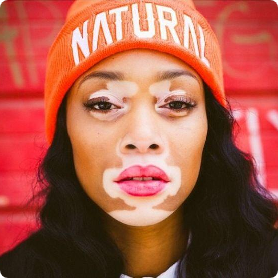The image is a close-up of a woman with long, dark hair, who is looking directly at the camera. She is wearing an orange woven beanie with the text "Natural" embroidered on it. Her skin is of a darker tone, but she has noticeable white patches around her eyes, lips, and chin, indicative of vitiligo. Her eyelashes are long and thin, and she is wearing bright pink lipstick. She is dressed in a black coat over a white t-shirt. The background of the image features pinkish-red hues, but her face and head dominate the composition.